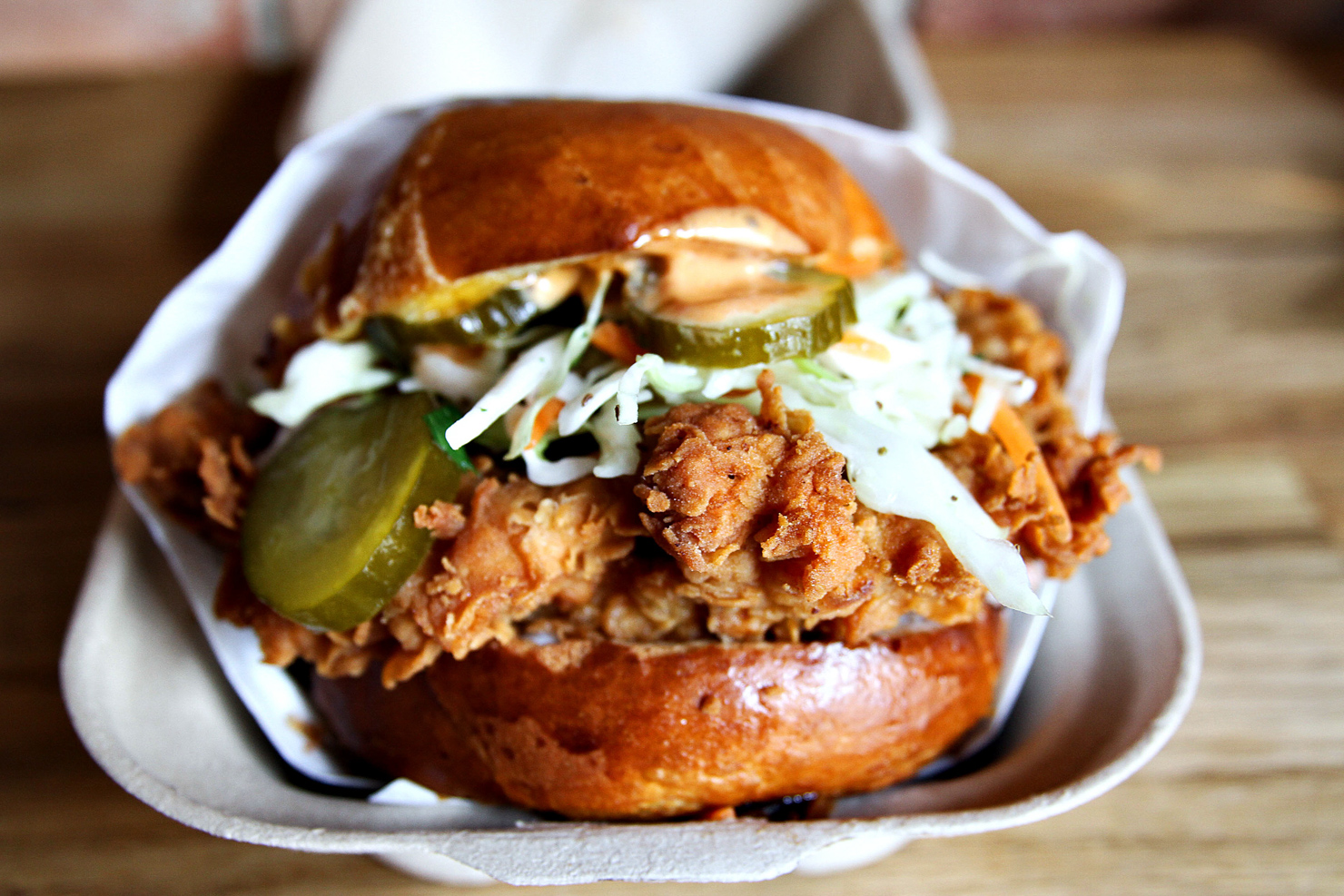This photograph showcases a golden-brown, perfectly glazed bun, highlighting a hearty and appetizing fried chicken sandwich. The sandwich is nestled in a paper sleeve, placed within an open, clamshell paper takeaway container set on a wooden surface. The bun, round and shiny, encases a generous piece of fried chicken, whose crispy breadcrumb batter sports a deep golden hue. The fried chicken overflows beyond the bun, emphasizing its substantial size. On top of the chicken lies a fresh layer of coleslaw, accompanied by sliced pickles and a slice of yellow cheese, adding vibrant contrast and texture to the dish. The overall presentation promises a delightful culinary experience.